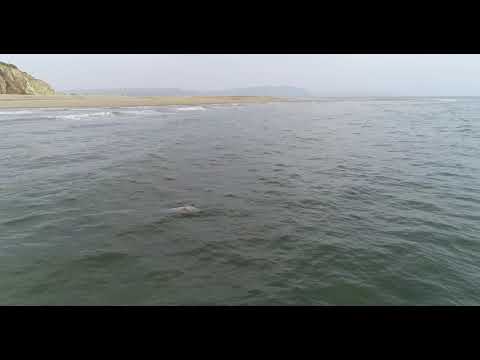The image captures a serene oceanscape on a gray, overcast day, suggesting perhaps an early morning or pre-storm atmosphere. The foreground is dominated by calm, sea foam green water, with small waves and white caps visible as they approach a deserted brownish-beige sand beach. To the left, a small sandbar or beach extends into the water, flanked by a subtle mountainous rock formation. In the distance, shrouded in a light mist, a larger mountain or island peaks through, adding depth to the scene. The beach area appears utterly deserted, with no people or structures in sight, enhancing the sense of tranquility and isolation. There seems to be an indistinct object in the water near the foreground—a dark lump that could be a sea turtle, a fish, floating debris, or possibly even a jellyfish—adding a touch of mystery to the otherwise calm and desolate scene.